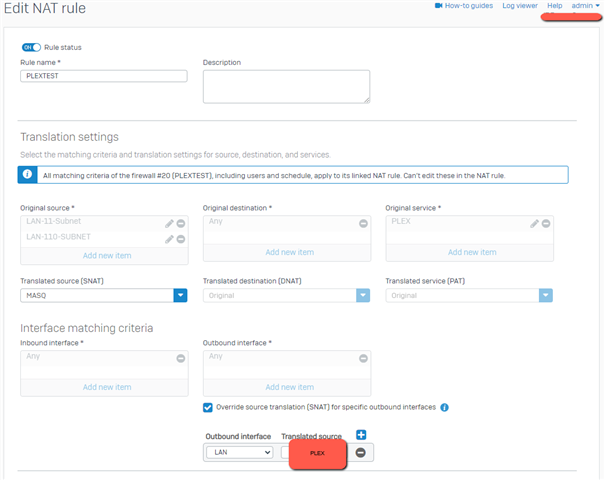This is a detailed screenshot of the "Edit NAT Rules" section from a website's administrative panel. In the top right corner, the word "admin" is displayed, with the associated username obscured by a red stripe to maintain privacy. At the bottom center of the screenshot, there are two options: "Outbound Interface" on the left, featuring a drop-down menu currently set to "LAN," and "Translated Source" on the right, which is highlighted by a red box that has been edited into the image. Inside this red box, the text "Plex" (P-L-E-X) is clearly indicated, suggesting that the user should input the name "Plex" into the "Trusted Source" field.

At the very top of the image, on the left side, a toggle switch is visibly set to "on." Adjacent to this switch, the label reads "Rule Status." Directly below this, there is a field named "Rule Name," which is filled out with "Plex test." To the right of the "Rule Name" field is an empty, large text box designated for a description.

The section underneath is titled "Translation Settings." Here, an info box provides additional context: "All matching criteria of the firewall number 20 Plex test, including users and schedule, apply to its linked NAT rule. Can't edit these in NAT rule." This info box explains the unmodifiable nature of certain settings, highlighting why the user took the screenshot to demonstrate the necessity of entering "Plex" in the "Trusted Source" field at the bottom of the panel.